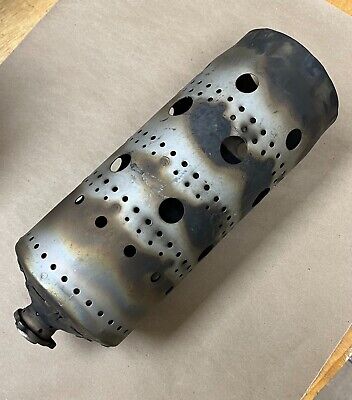The photograph depicts an old, silver cylinder with a pointed top capped with a gear-like structure. The cylinder, which appears to have burn marks and rusty ribbons, is lying sideways on a piece of brown paper against a wooden floor background. The surface of the cylinder is dotted with intricately and precisely made holes. There are several rows of these holes—two rows of small pinholes and one row of larger holes near the bottom. The sides of the cylinder, full of these blackened, burnt holes, suggest significant wear and damage.